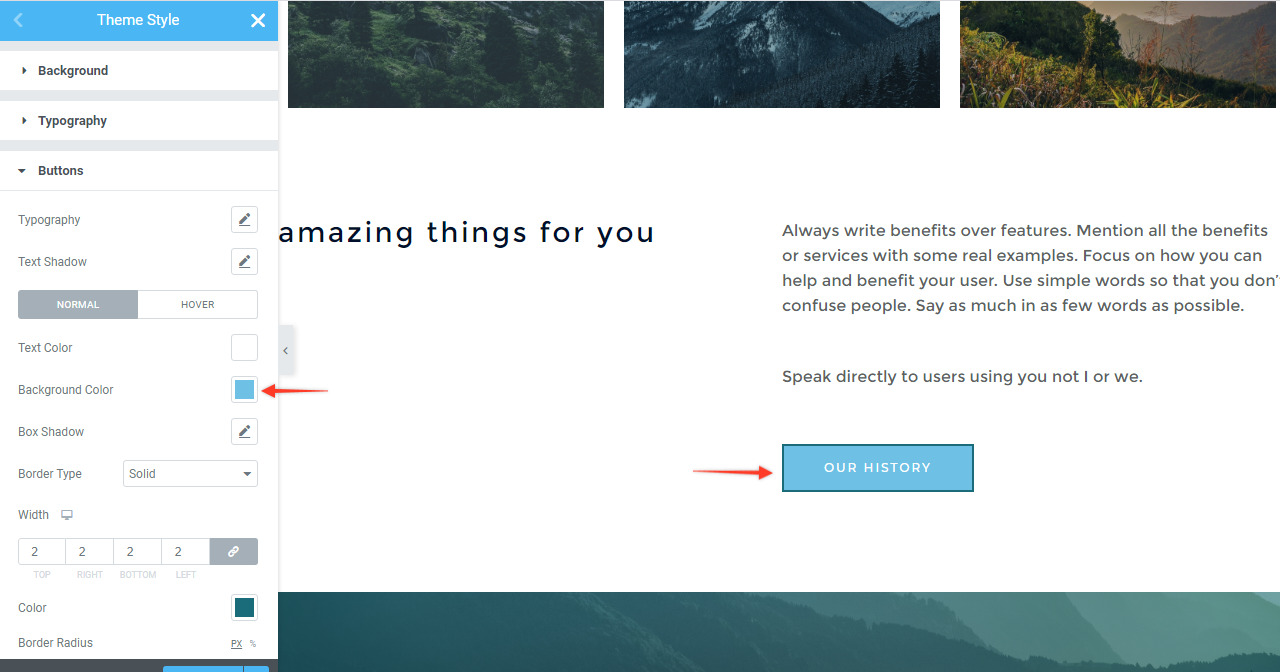The image displays a user interface with three partially cut-off rectangular photographs centrally positioned at the top. The first picture on the right showcases a picturesque grass field in shades of yellow-green and orange, set against a backdrop of towering mountains. To its left, the second image provides an aerial view of a forest bathed in a striking blue tint. The third image on the far left, with a greenish hue and a touch of fog, depicts green trees merging into a broad grassy landscape.

In the top left corner of the interface, the phrase "Theme Style" is prominently displayed, alongside a left-pointing arrow. Below this section, a list of categories appears, each paired with an arrow. The categories "Background" and "Typography" have arrows pointing to the right, suggesting submenus or collapse options, whereas "Buttons" has a downward arrow indicating an expanded view. Further down, additional categories are listed: "Typography," "Test Status," "Test Order," "Background Color," and "Back Slideshow," suggesting functional elements or further organizational settings within the interface.